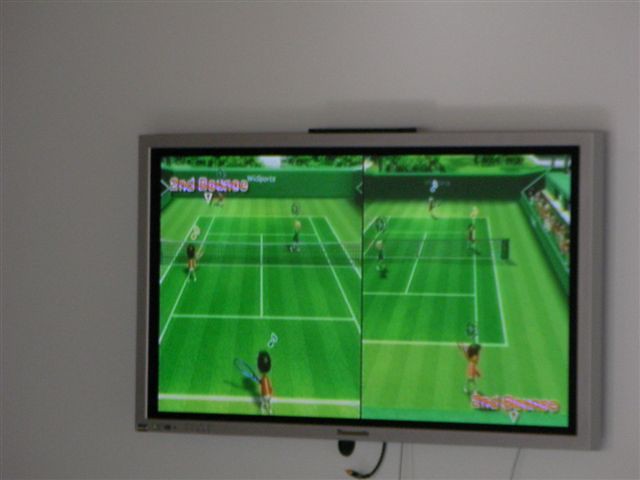The image depicts a small television mounted on the wall, displaying a split-screen setup. The screen shows a video game, specifically Wii Sports Tennis, with two separate in-game perspectives side by side. Each side of the split screen represents one player's view in the match, competing against each other. While it is difficult to discern all the text, it appears to indicate the "second round". Both sides of the split screen show four characters, implying a doubles match is taking place in the game. The setting and format make it clear that the players are engaged in a competitive session of Wii Sports Tennis.